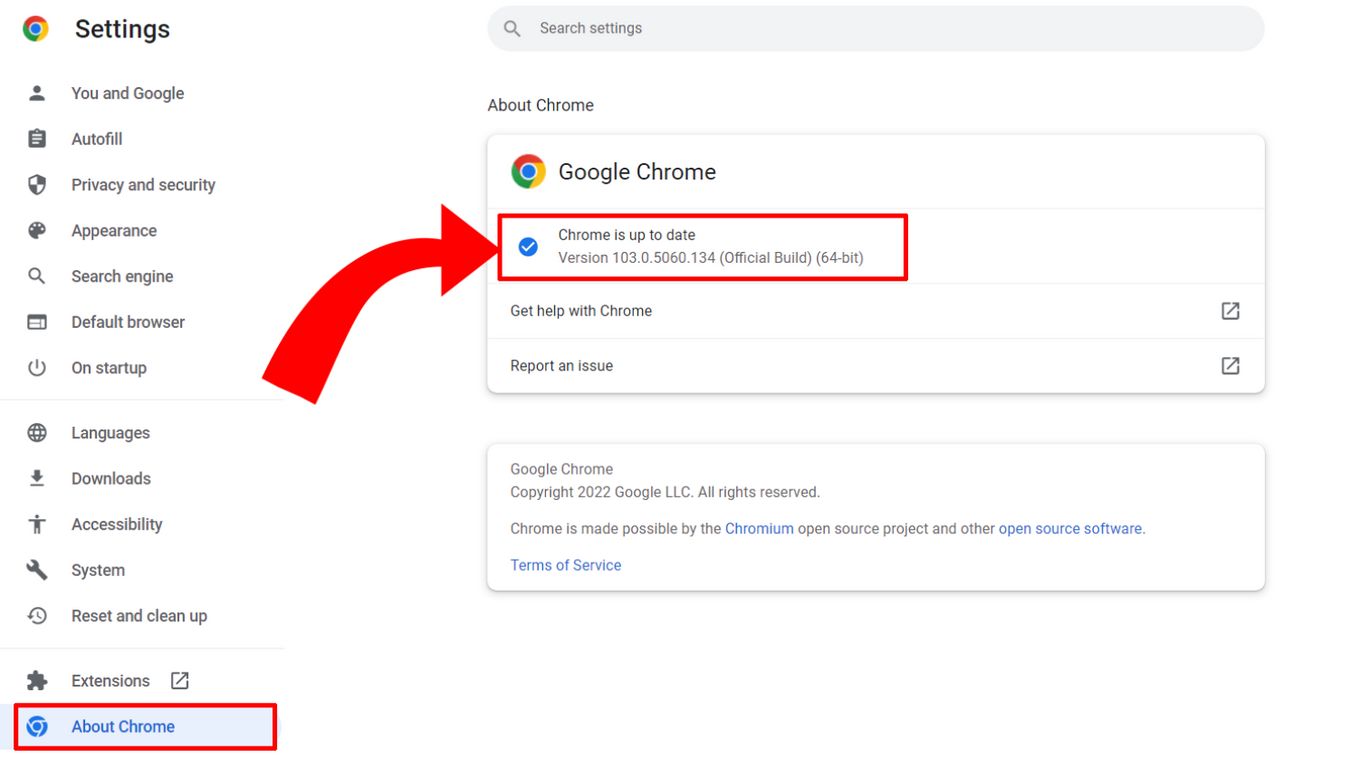This is a detailed screenshot of the Google Chrome Settings page on what appears to be a laptop or desktop computer, though it could also be a tablet in landscape mode. The top left corner displays the Google Chrome icon accompanied by the word "Settings" in bold, with a capital 'S' and the remaining letters in small caps. Situated at the top right is a search bar for navigating settings.

The "About Chrome" section is highlighted in the navigation pane, which is marked by a distinct red text box. The navigation pane on the left lists various settings categories: "You and Google," "Autofill," "Privacy and Security," "Appearance," "Search Engine," "Default Browser," "On Startup," "Languages," "Downloads," "Accessibility," "System," "Reset and Cleanup," "Extensions," followed by the currently selected "About Chrome."

On the right side of the screen, the "About Chrome" section provides key information. It confirms that "Chrome is up to date," along with the version number. A thick red arrow points to this status, which is emphasized with a red outline and a blue checkmark to its left. Below this, there are options to "Get Help with Chrome" and "Report an Issue," followed by Google's copyright information.